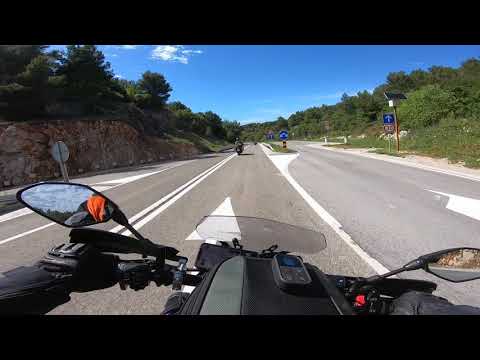The image appears to be taken from the perspective of a motorcyclist, possibly within a computer game due to its slightly animated feel. It depicts a two-lane road on a clear day, with the handlebars, rider’s hands, speedometer, and rearview mirror visible in the foreground. Approximately 40 feet ahead, another motorcyclist riding an all-black motorcycle is seen. The road surface is light brown asphalt with a white arrow pointing forward painted directly in front of the rider, and a double white line marking the left boundary. To the right of the primary lane, there's a pull-off area demarcated by additional white lines. Lush trees and greenery line both sides of the road, with a stone wall to the left and a small hill covered with trees. Among the roadside elements, there are blue signs; one featuring an arrow and a noticeable solar panel, suggesting it is solar-powered. A round sign sits to the left, alongside diverse roadside landscaping. The sky is mostly clear, with a solitary cloud near the top of the image.